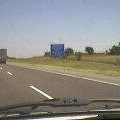This extremely small and grainy square-shaped photograph is captured from the perspective of a vehicle's dashcam or front seats, looking out through the front windshield. The scene is framed by the black edges of the car's windshield at the bottom of the image. The road ahead is a gray two-lane freeway marked by dotted white center lines and a solid white edge border line. A truck is visible ahead on the road, partially showing both its back and front. Surrounding the road is a flat green field, dotted with small green trees. The backdrop features a clear blue sky with no clouds. In the distance on the right side, a blue road sign with white text can be seen, though the text is unreadable due to the photo's graininess. The windshield wiper of the car is also visible, emphasizing the interior viewpoint from which this daytime scene is captured.